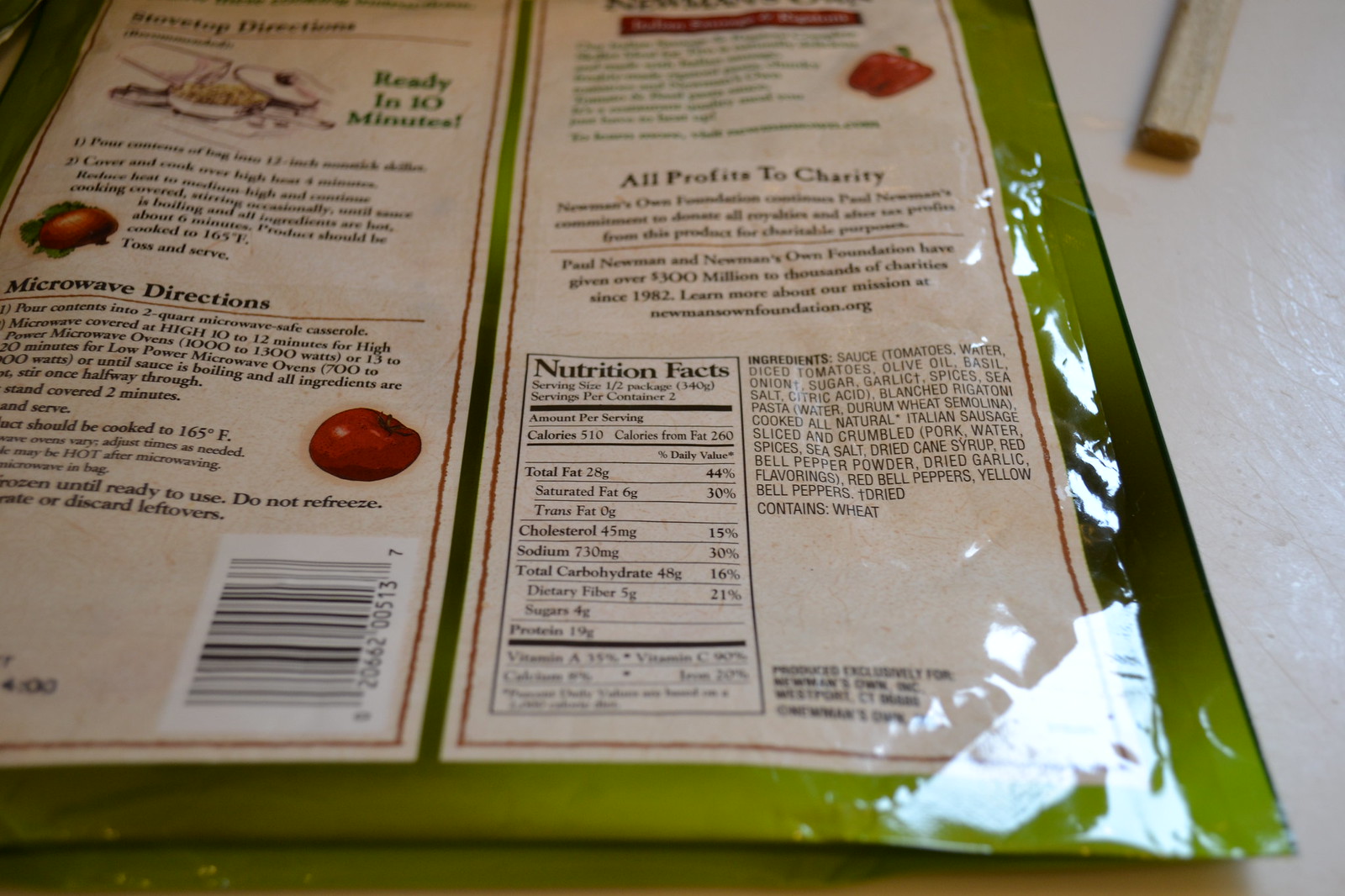The photograph captures a food package placed face down on a white surface, revealing its back side. The packaging is a soft, light pea-colored green material featuring beige labels. Positioned in the top left, stove top directions are outlined, indicating "ready in 10 minutes" with an illustration of a pan. Adjacent to this are microwave directions. Various graphical elements adorn the package, including illustrations of a tomato, a red bell pepper, an onion, and other vegetables, implying a tomato-based food product. Prominently displayed in the top center, the text "all profits to charity, Newman's Own Foundation" is visible, although partly obscured. Below, the nutrition facts and ingredient list are clearly printed in black font. The photograph also captures the end of a chopstick in the top right corner of the frame.